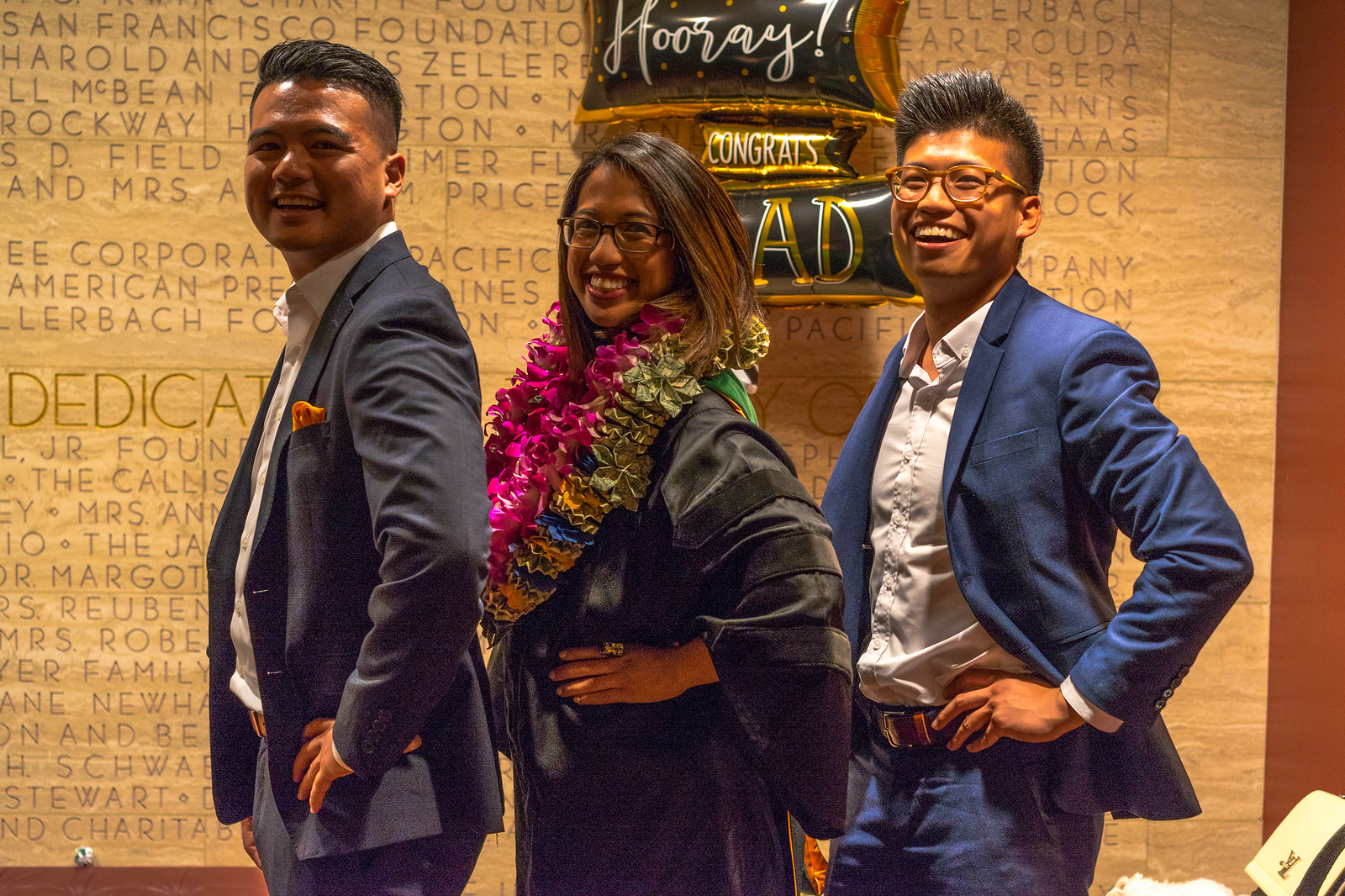The image depicts a celebration scene featuring three well-dressed individuals of Asian descent, standing in the center, directly posing for the camera against an indoor backdrop that includes a large, partially obscured poster with some text and celebratory balloons that read "hooray" and "congrats." The individuals appear to be at a graduation event, as suggested by the woman's attire and accessories. The man on the left wears a grey suit with a white dress shirt and an orange pocket square, and he is smiling. The woman in the middle, donning black graduation robes and multiple colorful flower leis around her neck, has brown hair and glasses. The man on the right sports a blue suit, blue pants, and yellow glasses, paired with a light blue dress shirt. The background features a decorative wall with engravings, adding to the celebratory atmosphere. The variety of colors present in the scene—including tan, brown, black, gray, orange, purple, pink, blue, green, and yellow—contribute to the festive setting, which may possibly be in Hawaii given the traditional Hawaiian leis worn by the woman.